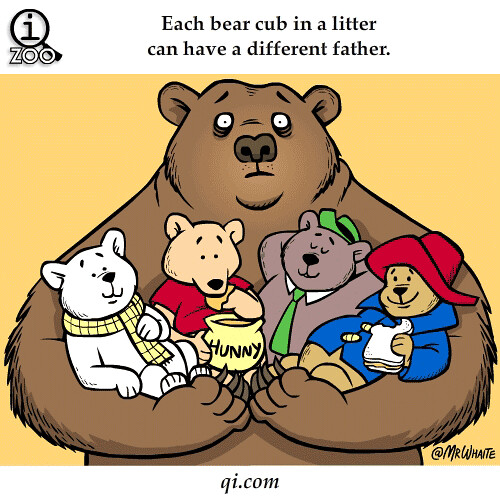This image is a comic book-style illustration with a yellow background. In the upper left corner, there is a magnifying glass with an eye in it, with the word "zoo" beneath it. Below this, the text reads, "Each bear cub in a litter can have a different father." Below this text, a large brown bear stands with its arms open, holding four smaller bears. 

The first small bear is a white polar bear with a tan checkerboard scarf, resembling the Coca-Cola Bear. The second is a light brown bear that looks like Pooh Bear, dressed in a red shirt and holding a pot labeled "H-U-N-N-Y." The third bear is dark black with a green hat and tie, resembling Smokey the Bear. The fourth bear is a brown bear dressed like Paddington Bear, wearing a red hat and blue coat, and eating a sandwich.

The bear family represents the idea that cubs in a single litter can have different fathers, depicted through the various well-known bear characters.